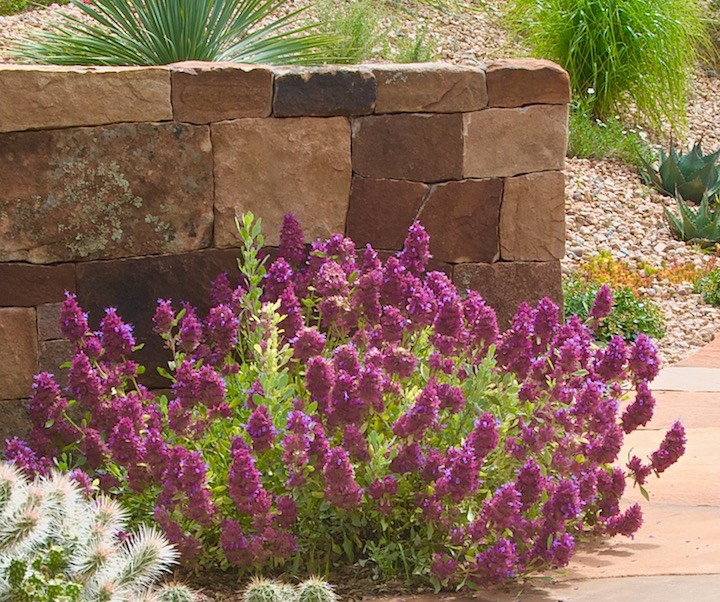The image captures an outdoor desert garden scene, prominently featuring a brown and tan brick wall adorned with patches of moss. In the foreground, vibrant purple flowers and prickly white blooms are depicted, adding a burst of color to the arid landscape. To the right, a barely visible tan sidewalk edges into the frame. Behind the stone wall, the ground is covered with small gravel stones, and there's an array of desert vegetation, including green, pokey plants and some orange-yellowish flora. The composition blends the rugged beauty of desert flora with the charm of a well-maintained garden. There is no text in the picture.